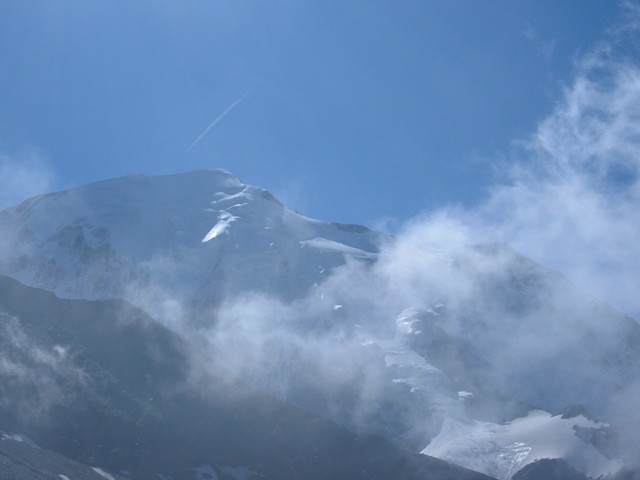The image showcases a vibrant blue sky adorned with an array of clouds, some of which exhibit a unique circular motion, suggesting the early formation of a tornado to the left. In the backdrop, there are three distinct mountain ranges; the farthest range is covered in snow, presenting a stark contrast to the nearer, minimally snow-capped mountain to the left. The right center also reveals snow-covered peaks amidst a foggy and cloudy atmosphere. The clouds gather and rise upwards to the right, creating an interplay of light and shadow over the rugged landscape, and hinting at a prehistoric figure formed by the cloud formations and rocky surfaces.